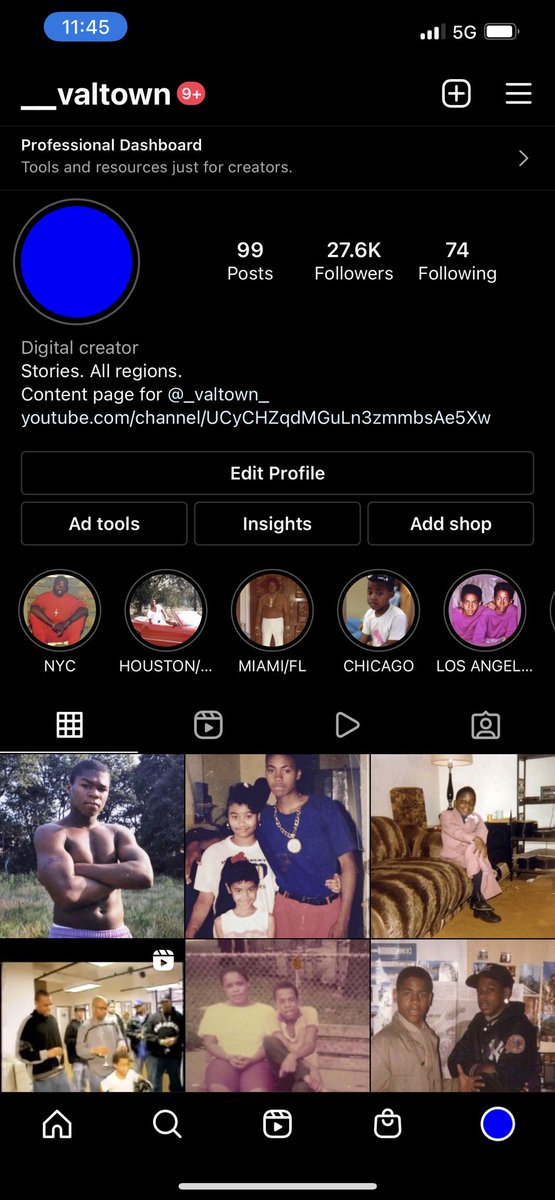This image captures a smartphone screen viewed in portrait orientation. The screen is rectangular, with a height twice its width, set against a solid black background. At the top of the screen, a blue oval-shaped bubble displays the time as "11:45" in white font. Adjacent to it on the right, a cellular network indicator shows 3 out of 4 bars with a 5G connection and a nearly full battery icon.

Beneath this status bar, the username "_VALTOWN" appears in white text, accompanied by a red notification bubble indicating "9+" new notifications. Below the username, there's an option to access the professional dashboard, which is signified by a blue circle icon containing text that states "99 posts, 27.6K followers, following 74."

The bio section identifies the account holder as a "Digital Creator" with a description that includes "Stories, All Religion, Content page for VALTOWN" and a link to a YouTube channel. Below the bio are story highlights labeled with locations: "New York City," "Houston," "Miami Florida," "Chicago," and "Los Angeles."

Further down, navigation options for viewing pictures, videos, and stories are presented. The main section of the screen displays six photos, predominantly featuring various families, suggesting a media page managed by the same individual.